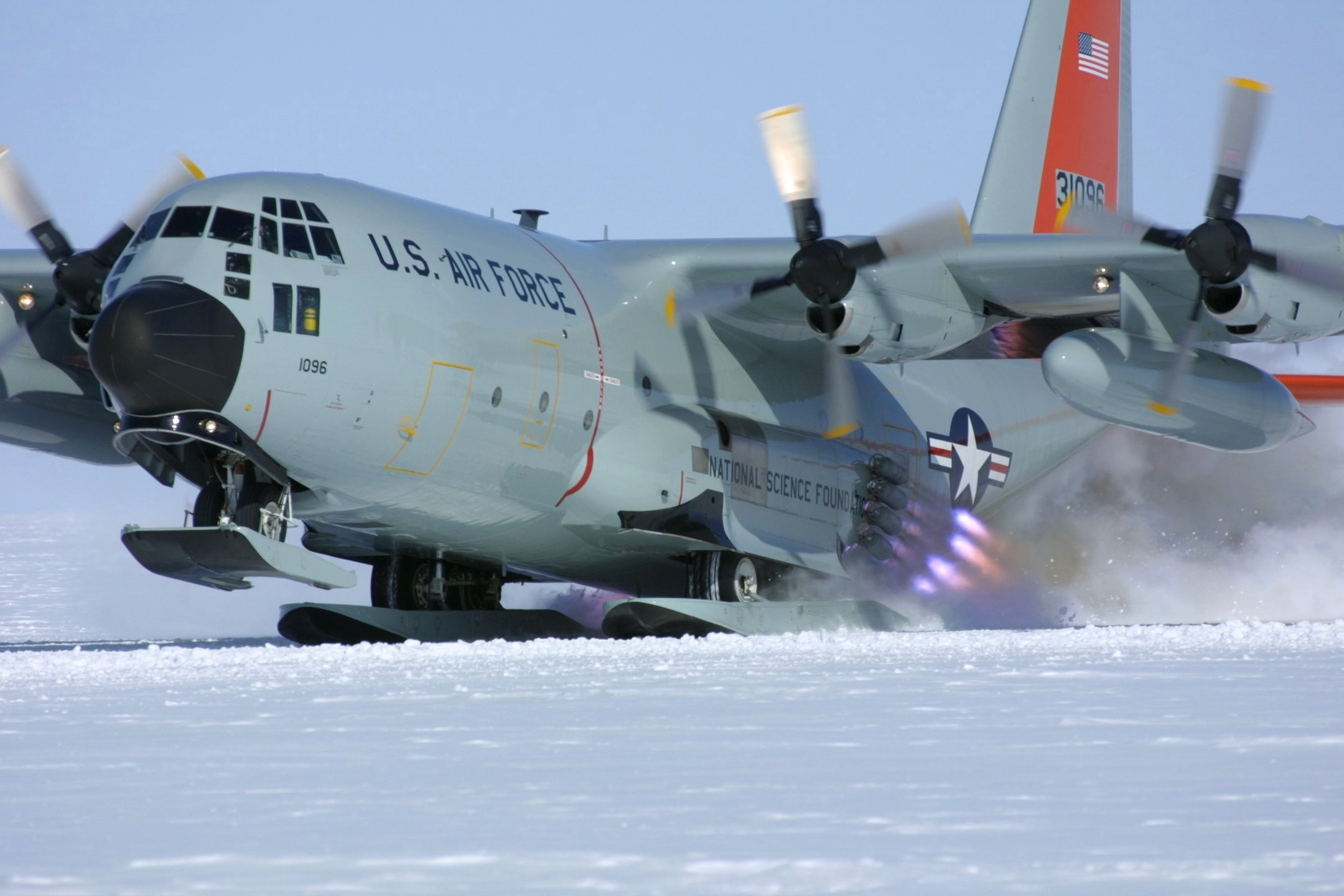This photograph captures a U.S. Air Force aircraft adorned in a gray livery. The plane is a four-propeller model, though only three propellers are visible in this image. The right wing displays its two propellers clearly, while the left wing reveals just one, with the remaining part of the wing extending out of view. The aircraft is equipped with skis for landing on snowy terrain and has touched down on a snow-covered area. Behind the right-side propellers, snow or possibly exhaust smoke can be seen swirling in the air. 

Prominently featured on the fuselage is a white star encircled by a blue background and flanked by red, white, and blue stripes. The aircraft's tail fin is marked by a red horizontal stripe against the gray backdrop, and it prominently displays an American flag alongside the identification number "31095." The underside of the aircraft bears the partially visible inscription "National Science Foundation," though only "FOUND" is clearly readable. Towards the front, the dark blue letters spell "U.S. Air Force" near the cockpit area, which is fitted with multiple windows typical of the cockpit's design.